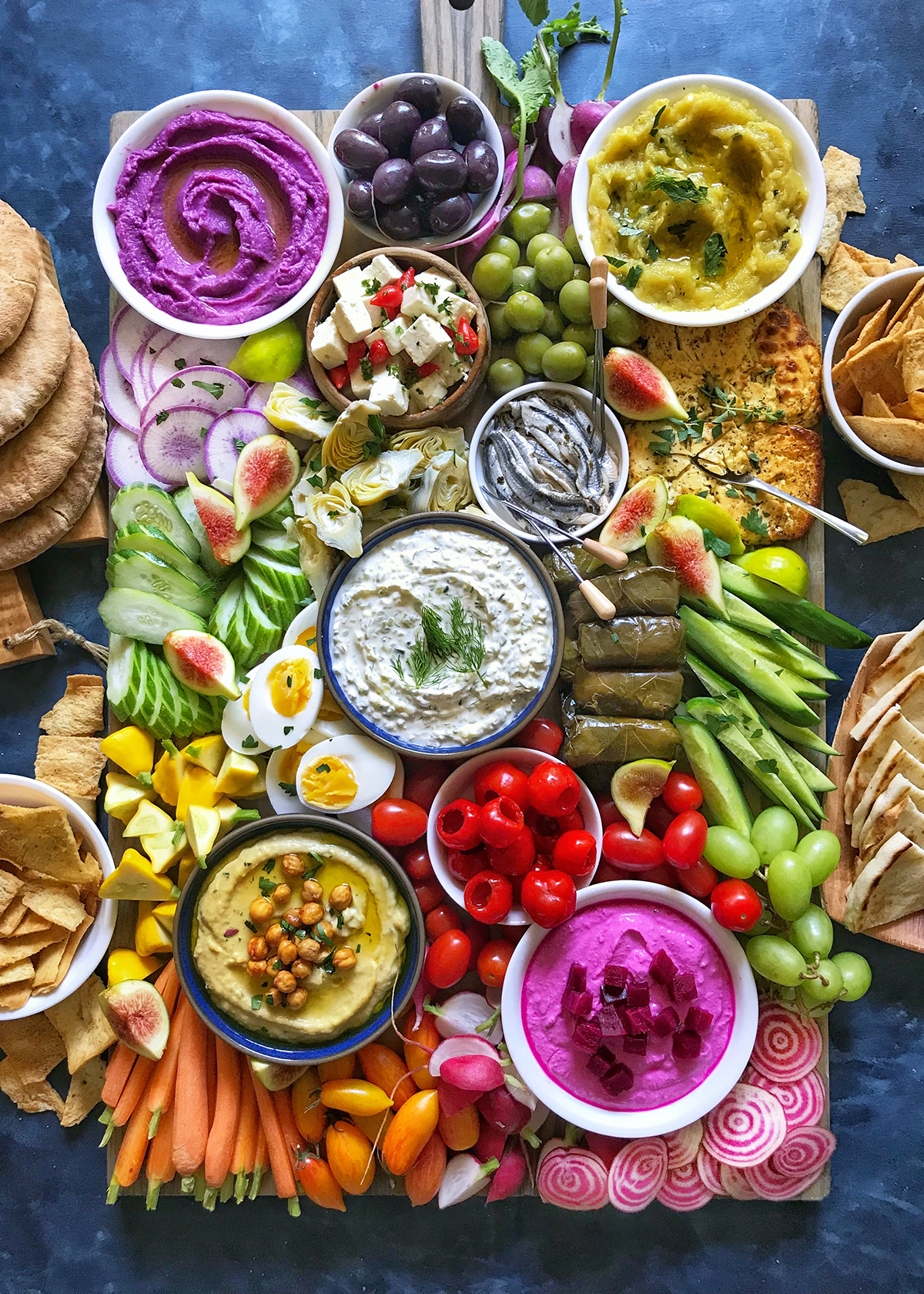This overhead color photograph captures an elaborate Mediterranean-style hors d'oeuvres platter artfully arranged on a rectangular wooden board, set atop a blue marble surface. The wooden board is densely packed with a wide variety of fruits, vegetables, dips, and snacks, creating a vibrant mosaic of colors and textures. In the top left corner sits a white porcelain container holding a purple dip, possibly a root vegetable puree. Adjacent to it are two small bowls, one with black olives and the other with green olives. Moving right, a yellow bowl contains hummus, flanked by a container of couscous garnished with green herbs and a bowl of what appears to be feta cheese mixed with tomato. 

Slices of toasted flan bread and pita chips are scattered about, complemented by bowls of crackers situated on both the left and right sides of the board. Sliced figs, cherry tomatoes, and pitted cherries add bursts of color throughout, while baby carrots, hard-boiled egg slices, and thinly sliced red radishes contribute fresh, crisp elements. In the bottom center lies a richly garnished purple dip, likely beets, with neighboring bowls containing what could be salsa or another type of dip. Stuffed grape leaves and occasional pieces of bread further enrich this smorgasbord, making it a feast for both the eyes and palate. Surrounding the board on the blue surface are scattered chips and other snack items, adding to the inviting, abundant display.